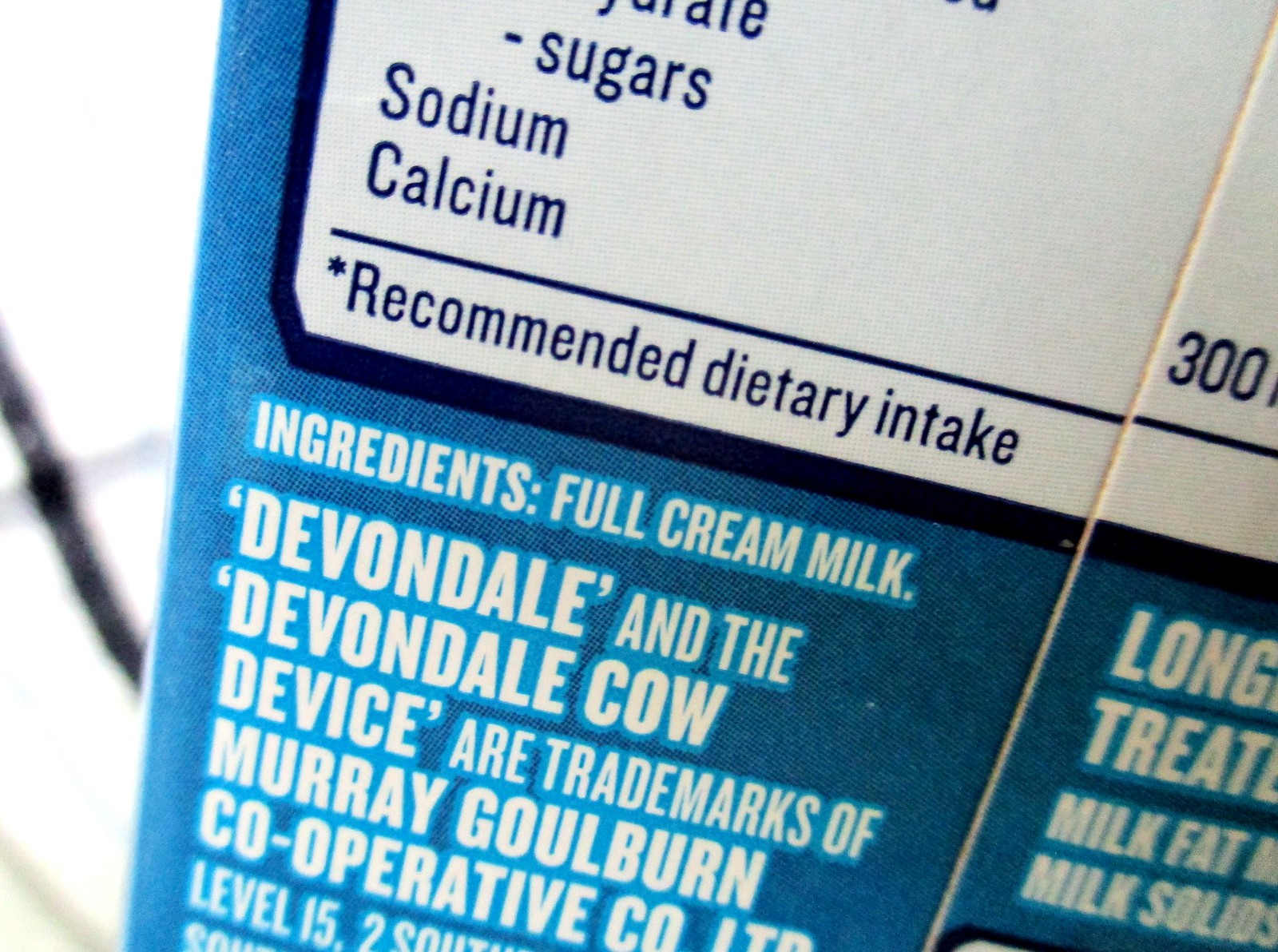The image is a close-up of a blue milk carton, tilted slightly to the right, set against a white surface with a black wire running along it. The carton features a white box with blue text at the top, bordered by a dark black frame. Inside this box, the text reads: “sugars, sodium, calcium,” followed by a partially visible “300” and “recommended daily dietary intake” with an asterisk, indicating a reference to specific dietary values. Below this, and partially cut off by the edges of the photograph, is a detailed ingredients list in white text with blue borders on the blue portion of the carton. The readable text includes: “ingredients, full cream milk, and the Devondale cow device are trademarks of Murray-Goulburn Co-operative Co Ltd, Level 15.” Further down, fragmented words such as “long treated milk fat” and “milk solids” are visible. The detailed text and design elements suggest this is the back label of the carton, providing nutritional and branding information.